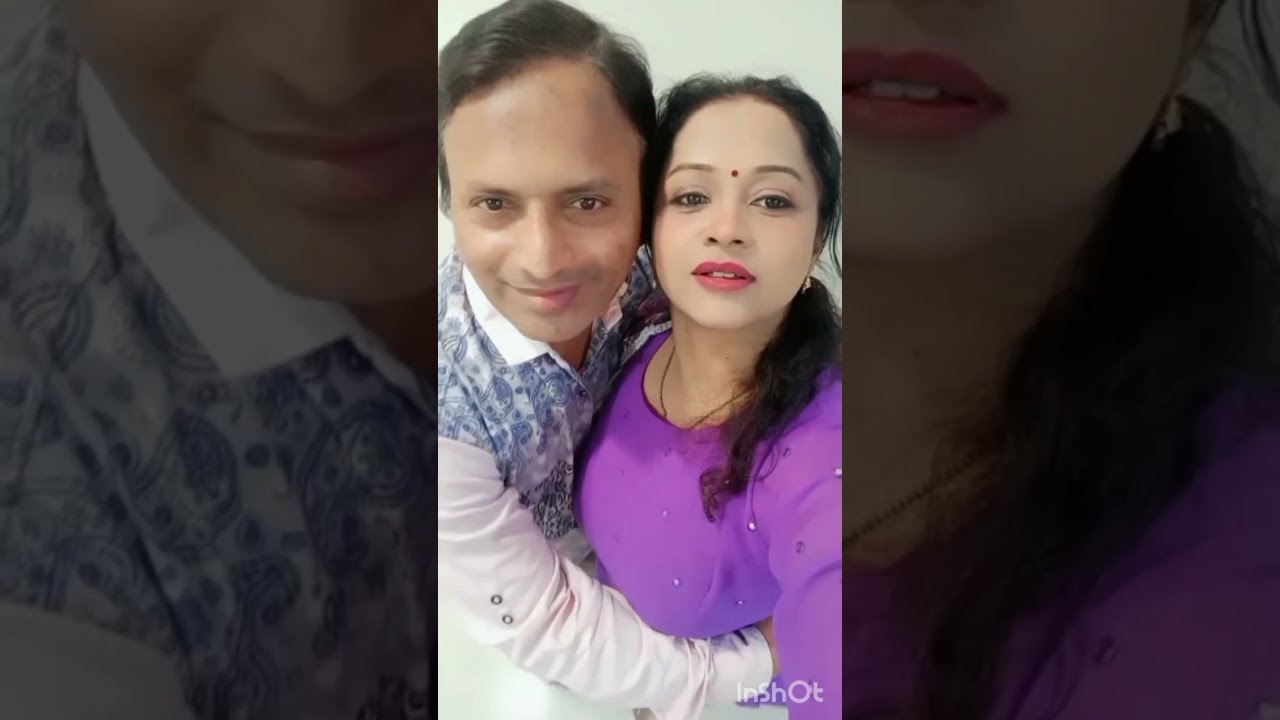The image features an embracing couple of likely Indian or South Asian descent, positioned centrally within a photograph divided into three vertical panels. The middle panel showcases the couple in full brightness, contrasting with the darker, shaded close-up views of their mouths on the left and right panels. The man, with short black hair and light brown skin, is on the left. He wears a white long-sleeve collared shirt adorned with a navy blue paisley pattern, resembling a vest. The woman, to his right, has dark brown hair tied in a ponytail and sports a red bindi on her forehead, along with red lipstick. She is dressed in a bright purple long-sleeve top embellished with small white gemstones that sparkle. Additionally, she wears a necklace. Both individuals have their eyes open and are smiling gently. The background is a simple cream or white, providing a neutral setting. The text "INSHOT" appears at the bottom right of the central panel. The overall atmosphere suggests a warm and intimate moment captured in a well-lit room.